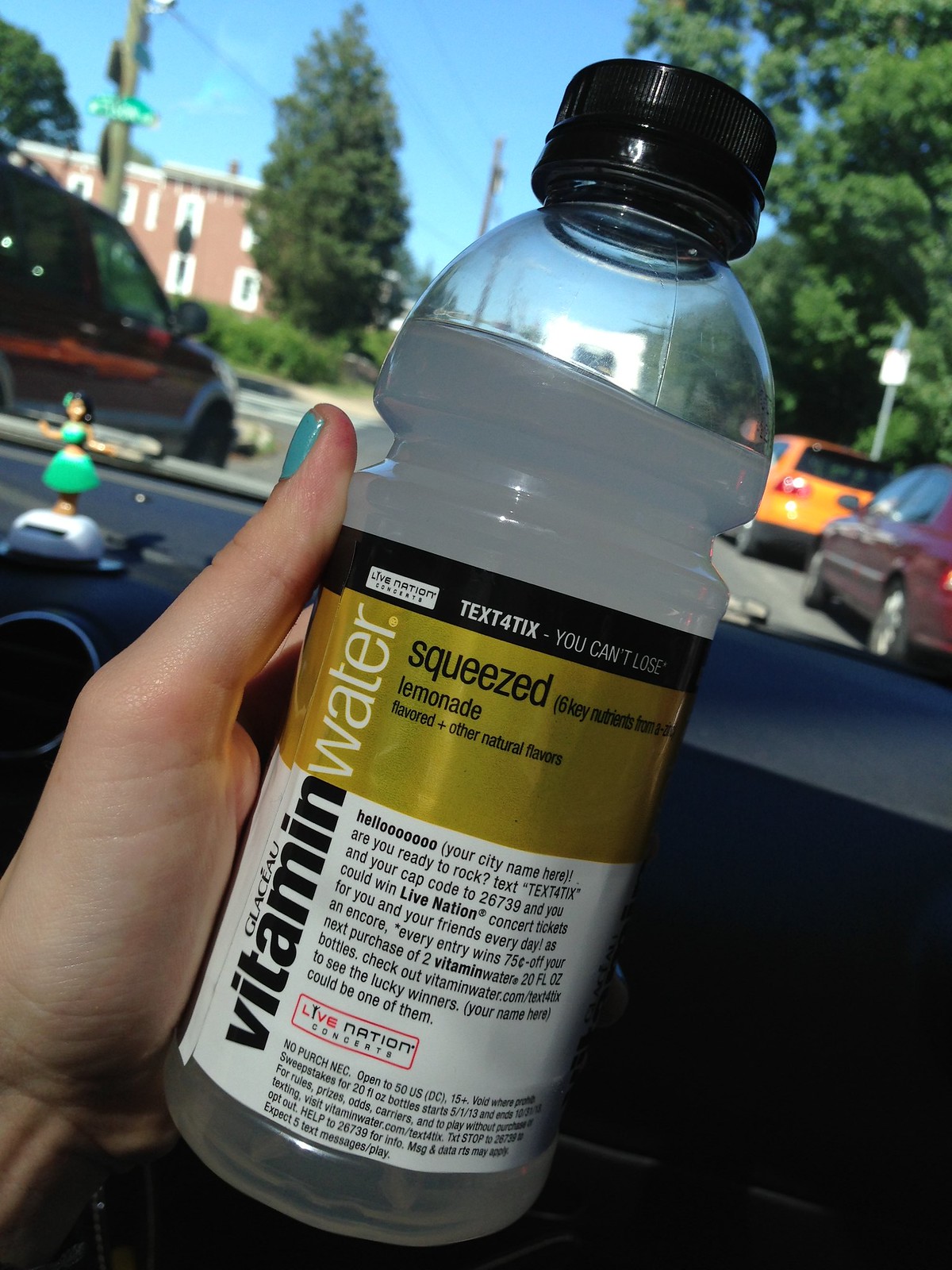In this vibrant color photograph, we see a perspective from inside a car. A person with fair skin is holding a plastic bottle with a black cap in their left hand. Notably, their thumb is painted a striking turquoise. The bottle contains a milky, watery liquid and prominently features a colorful label.

The label is from a promotion by Live Nation Concerts and Vitamin Water. It includes various text details, among them, "Text for ticks you can’t lose." It identifies the drink as "Class 2 Vitamin Water" with "Squeezed Lemonade Flavored plus other natural flavors," and boasts "six key nutrients." It also reads, "Hello [your city name here], are you ready to rock?" encouraging participants to text a specified code to 26739 for a chance to win concert tickets from Live Nation.

The promotional text also mentions that every entry wins 75 cents off the next purchase of two Vitamin Water 20 fl oz bottles, inviting consumers to visit VitaminWater.com to check for winners. It lists terms and conditions, including a note that the promotion runs from May 1, 2013, to October 31, 2013, and is open to residents of the 50 US states and DC, aged 15 and up. Additional information on how to play without purchase, rules, and carrier-related queries can also be found on the label.

This photograph not only captures the product but also creatively informs about the promotional campaign in a detailed manner.